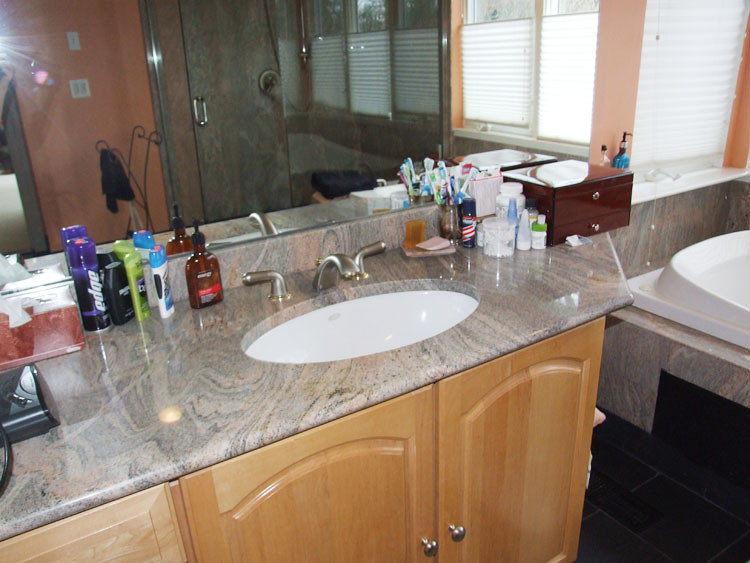The photograph captures a modern bathroom with a rectangular orientation, where the longer side extends horizontally. Prominently positioned in the center of the image is a countertop made of gray granite, equipped with a sink. To the far right of the image, one can see a portion of a bathtub, hinting at its presence without fully displaying it.

Above the countertop, there is a large mirror. A camera flash is visible in the reflection, indicating that the photo was taken from the upper left-hand side. The mirror also reflects a shower located on the opposing wall, further emphasizing the spacious layout of the bathroom. Both the reflected and non-reflected sections of the wall have a warm, orangish hue.

A window with white blinds is situated in the upper right corner of the image, just outside the mirror's frame, adding natural light to the room. The countertop is crowded with various personal care items, including shaving cream, deodorant, a tissue box, a possible jewelry box, toothbrushes, cologne, and hand soap. A mysterious device is located on the far left of the countertop, next to a bar of soap.

Below the countertop, light brown, maple-like cabinets offer storage space. The same gray granite used for the countertop also trims the bathtub and seems to be employed in the shower's design, creating a cohesive and stylish look throughout the bathroom.